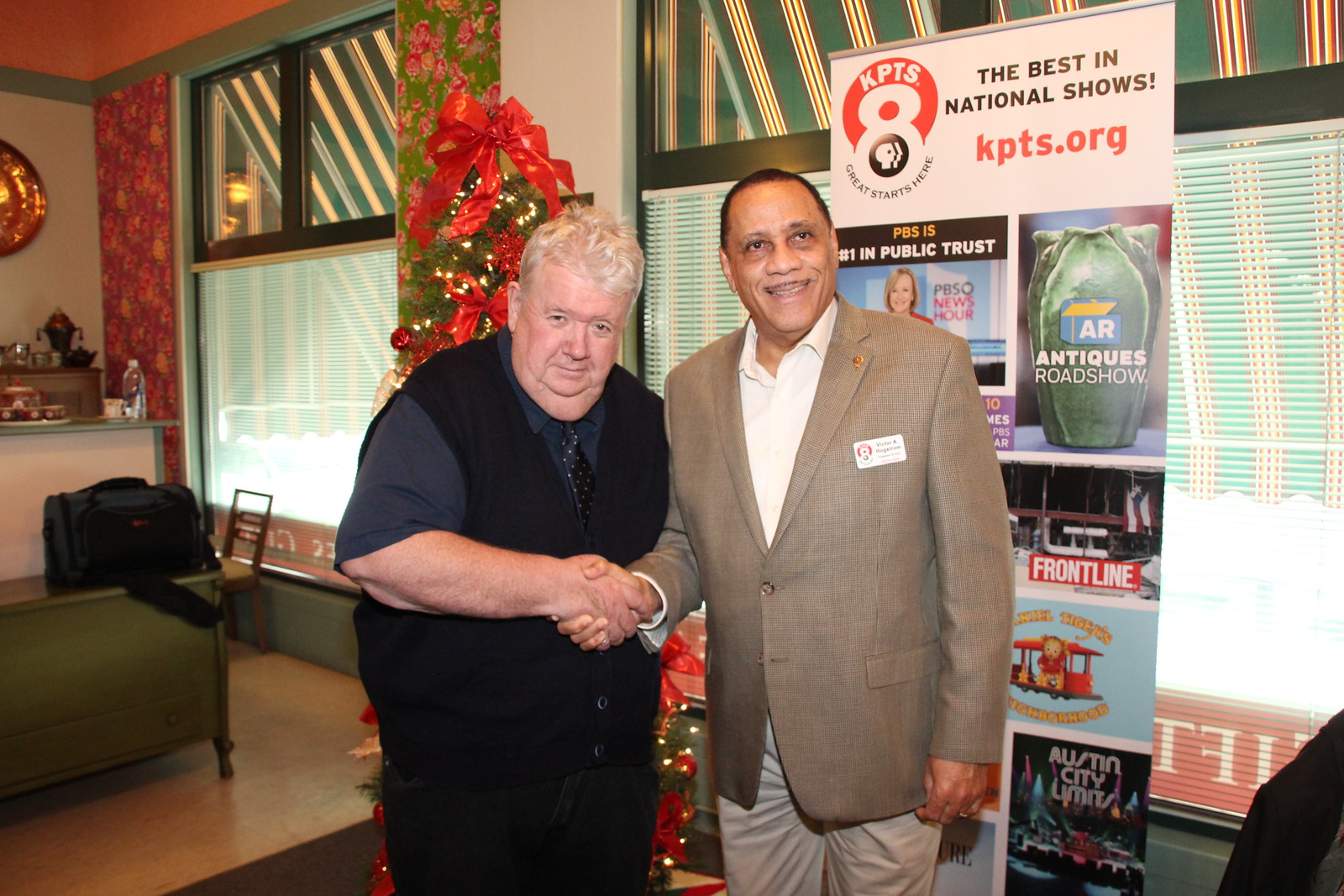In this image, we see two men shaking hands in what appears to be an office or a formal event setting. The man on the left, who seems older, is dressed in a black vest over a black shirt, paired with black trousers and a dark tie adorned with orange spots. The man on the right is in business casual attire, wearing a tan coat over a white collared shirt with tan trousers and a name badge. Behind them is a vertical banner displaying the text "The Best National Shows" along with the website kpts.org and a logo featuring "KPTS 8." This banner includes promotional content for shows such as Antiques Roadshow, PBS, Frontline, and Austin City Limits, indicating their association with a PBS-affiliated TV station. Additional details in the background include green window blinds, two windows, and a decorated Christmas tree, suggesting a festive atmosphere.